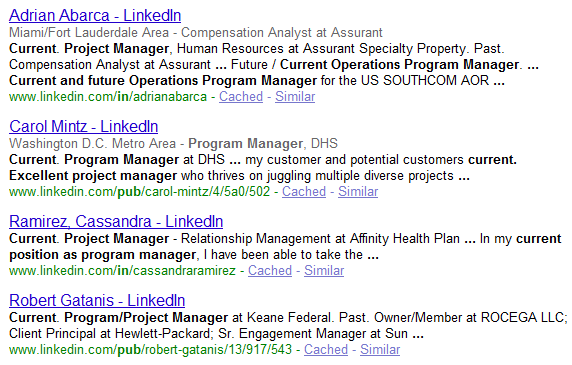The image displays a series of search results related to LinkedIn profiles. Each entry consists of hyperlinked titles in blue and additional details beneath.

1. **Adrian Abarca - LinkedIn**
   - _Location:_ Miami/Fort Lauderdale Area
   - _Current Position:_ Compensation Analyst at Assurance
   - _Previous Positions:_ 
     - Project Manager, Human Resources at Assurance Specialty Property
     - Compensation Analyst at Assurance
   - _Future/Current Roles:_ Operations Program Manager for the U.S. South Com A.O.R
   - _LinkedIn Profile URL:_ [www.linkedin.com/in/adrianabarca](www.linkedin.com/in/adrianabarca)
   - _Other Links:_ [Cache](link) | [Similar](link)

2. **Carol Mintz - LinkedIn**
   - _Location:_ Washington, D.C. Metro Area
   - _Current Position:_ Program Manager at DHS
   - _Current Role Description:_ Skilled in managing multiple diverse projects
   - _LinkedIn Profile URL:_ [www.linkedin.com/pub/carol-mintz/4/5A0/502](www.linkedin.com/pub/carol-mintz/4/5A0/502)
   - _Other Links:_ [Cache](link) | [Similar](link)

3. **Cassandra Ramirez - LinkedIn**
   - _Current Position:_ Project Manager - Relationship Management at Affinity Health
   - _Current Role Description:_ Extensive experience in program management
   - _LinkedIn Profile URL:_ [www.linkedin.com/in/cassandraramirez](www.linkedin.com/in/cassandraramirez)
   - _Other Links:_ [Cache](link) | [Similar](link)

4. **Robert Gattanis - LinkedIn**
   - _Current Position:_ Program Manager at Keen Federal
   - _Previous Positions:_ 
     - Owner/Member at Rocega LLC
     - Client Principal at Hewlett-Packard
     - Senior Engagement Manager at Sun
   - _LinkedIn Profile URL:_ [www.linkedin.com/pub/robert-gattanis/13/917/543](www.linkedin.com/pub/robert-gattanis/13/917/543)
   - _Other Links:_ [Cache](link) | [Similar](link)